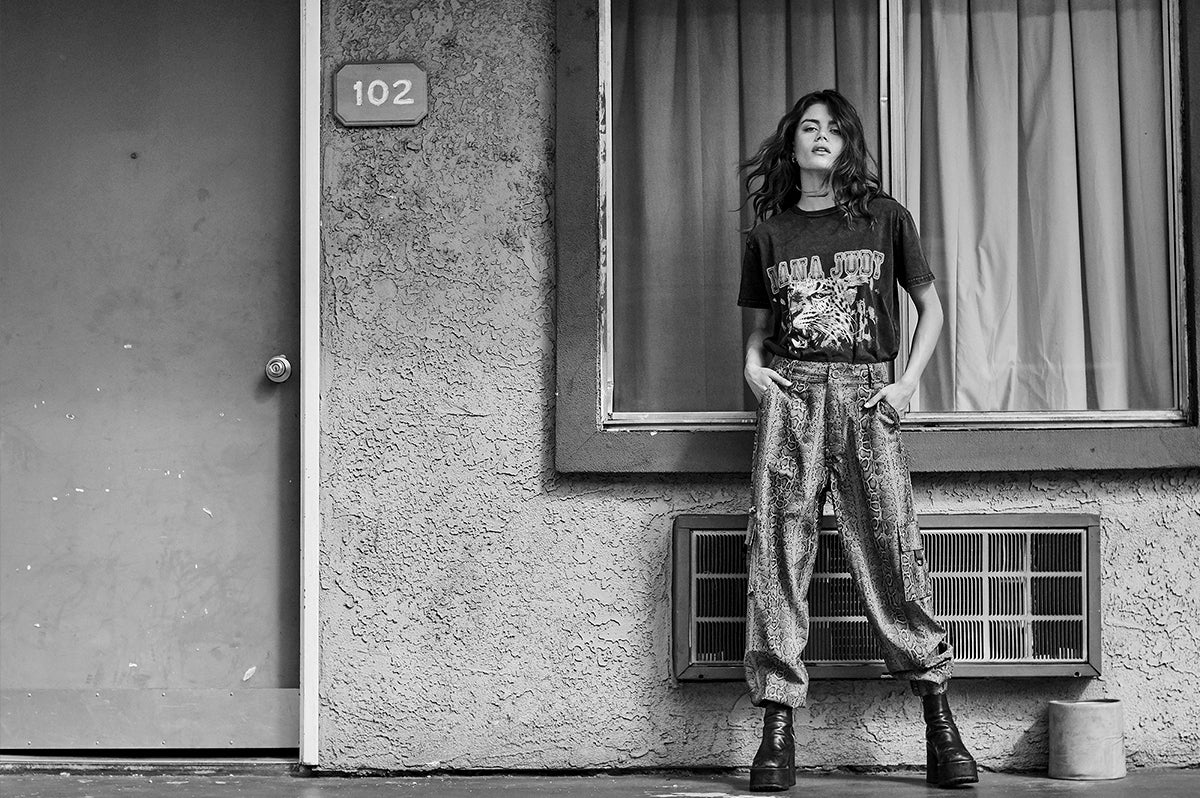This is a black and white, horizontally aligned, outdoor photograph of a young woman, likely in her 20s, standing in front of an old, textured, light stone building, possibly a motel. She stands confidently in front of a large window with curtains, positioned above air conditioning vents. Her hands are in the pockets of her baggy, patterned gray and white pants. She wears a black t-shirt with the text "Nana Judy" and a graphic of a cougar or leopard. Her long, wavy hair, either black or brown, cascades over her shoulders. She dons black combat boots and stands near a door marked with the number "102" and a silver doorknob. The ground beneath her appears to be concrete. Her head is slightly turned upward, giving her a sullen or defiant expression.